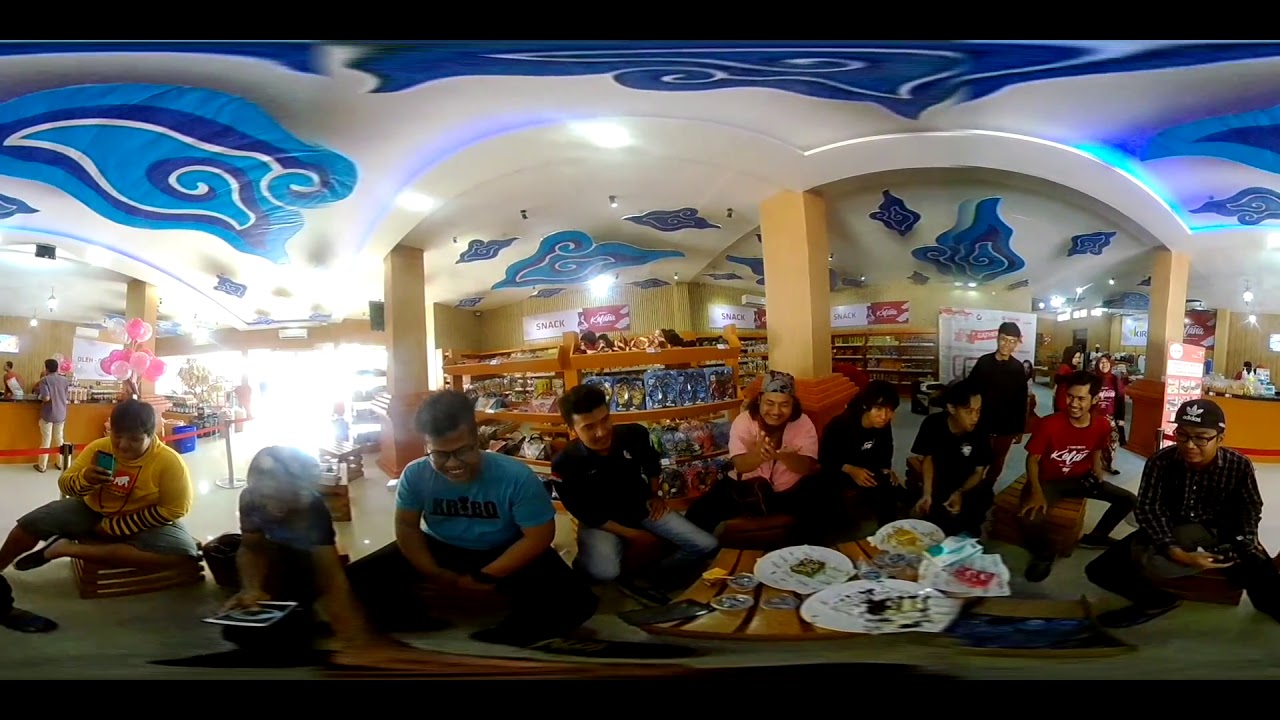The photograph captures a diverse group of people gathered around a large wooden table, decked with white plates and an assortment of food, suggesting a communal meal. The setting appears to be an indoor space, possibly a restaurant or store, characterized by its vibrant decor. Above them, the ceiling features intricate turquoise, royal blue, and white designs, adding a festive ambiance to the scene. 

The group displays a mix of colorful and casual clothing, with individuals wearing a yellow hoodie, a turquoise blue short-sleeved t-shirt, a black shirt, a light pink cardigan, a red short-sleeved t-shirt, a black collared checkered long-sleeved shirt, and various other outfits. A person in a gray shirt and white pants is seen standing near a counter, which is brown at the bottom and black at the top, suggesting a service area with roped-off sections.

Bookcases or shelving units line the background, filled with an assortment of items, adding to the impression of a bookstore or multi-purpose space. Pink balloons provide a festive touch on the left side of the image. The overall mood is lively and convivial, capturing a moment of shared enjoyment among the group in this richly decorated and bustling environment.